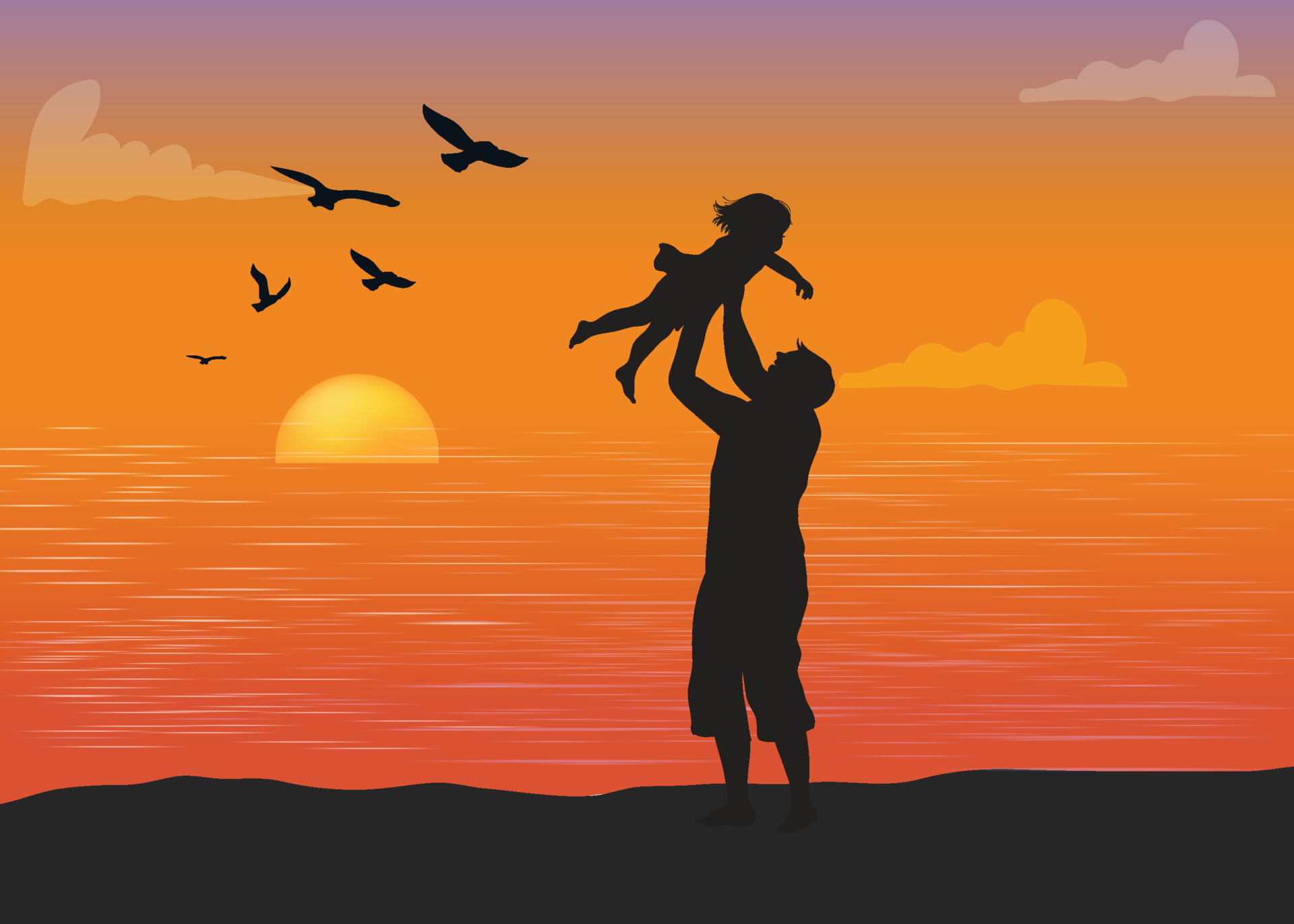The illustration depicts a joyful beach scene at sunset with a vibrant color palette transitioning from red to orange to pink, culminating in a warm yellow sun halfway submerged in the horizon. The background includes white, wispy clouds, while five silhouetted seabirds soar diagonally upward from the left. In the foreground, rendered entirely in black silhouette, a man stands just off-center with his legs partially rolled up, suggesting contact with the water. He joyfully lifts a young girl above his head, her hair and dress billowing in the wind, capturing a moment of playful delight. The scene is a striking interplay of warm sunset hues and stark black shadows, framed by subtle white lines that hint at the waves beneath.